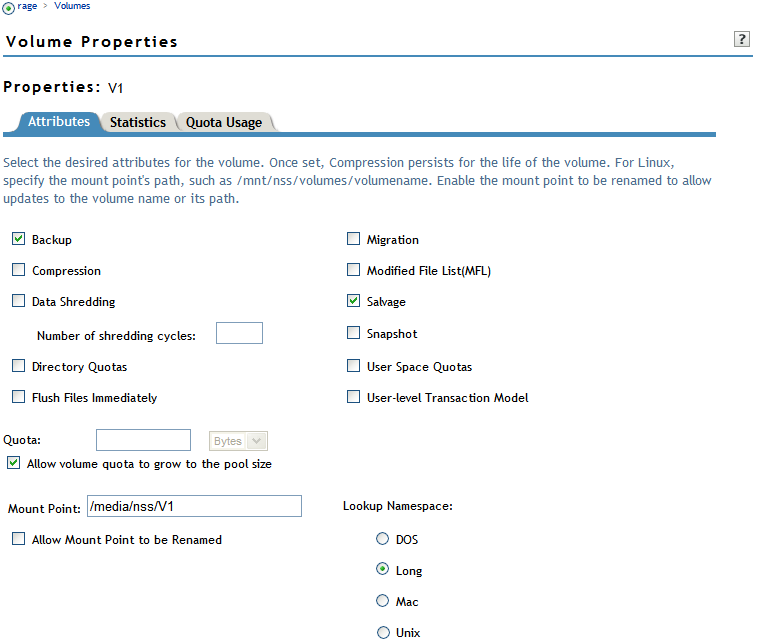This is a screenshot from an unidentified web page, prominently featuring a section dedicated to volume properties. The interface display is structured and somewhat technical, with blue lowercase text reading "rage" located in the top left corner. Adjacent to this, an arrow labeled "Volumes" points rightward, leading to "Volume Properties" and further specified as "Properties V1."

The interface is organized into three tabs: "Attributes" (the selected tab), "Statistics," and "Quota Usage." Within the "Attributes" tab, a detailed set of options and settings for volume management are displayed. 

The description includes guidance for selecting desired attributes for the volume and emphasizes that once compression is set, it remains effective for the volume's lifetime. For Linux systems, users are instructed to specify the mount point's path, citing an example format such as `/mnt/nss/volumes/volume_name`. Users also have the option to enable the mount point to be renamed, which facilitates updates to the volume name or its path.

Several checkboxes and settings are visible, indicating various attributes and capabilities:
- "Backup": Checked
- "Compression"
- "Data Shredding"
- "Number of Shredding Cycles"
- "Directory Quotas"
- "Flush Files Immediately"
- "Migration"
- "Modified File List (MFL)"
- "Salvage": Checked
- "Snapshot"
- "User Space Quotas"
- "User Level Transaction Model"
- "Quota": Checked, allowing volume quota growth to the pool size
- "Mount Point": Specified as `/media/nss/v1`
- "Allow Mount Point to be Renamed"
- "Lookup Namespace":
  - "DOS"
  - "Long": Checked
  - "Mac"
  - "Unix"

The layout and options suggest a comprehensive system for managing various aspects of volume properties, likely intended for users with some technical background in system administration or data management.